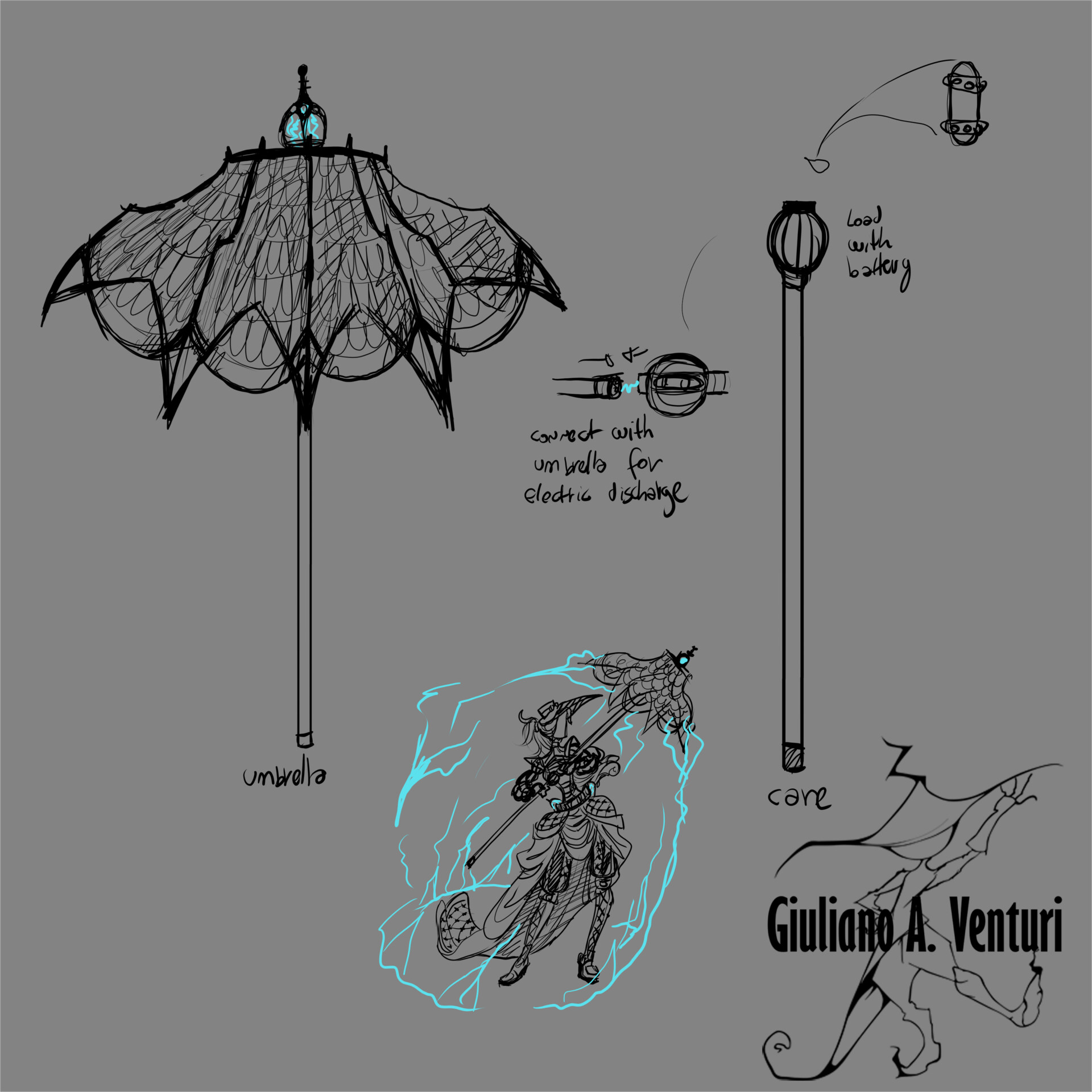This detailed and artistic illustration, set against a grey background, features several interconnected sketches primarily drawn in black. On the left side, there's a simple drawing of an umbrella, labeled "umbrella" below it. Adjacent to this umbrella, a depiction of two wires is shown with blue-colored electricity connecting them, accompanied by the text "connect with umbrella for electric discharge." On the right side of the composition, there's a sketch of a pole or cane topped with a hand lamp-like structure, labeled "load with battery," indicating a battery positioned on the upper right side. 

The center of the image features a prominently drawn woman in a long dress and hat, holding an umbrella surrounded by vivid blue lightning bolts, suggesting she is being shielded or affected by an electric current emanating from the umbrella. At the bottom right corner, there's an intriguing, alien-like character with the text "Guiliano e Venturi" written above, possibly indicating the artist or a signature logo. The cohesive theme throughout the artwork is enhanced by the consistent black sketches and the electrically charged motifs.